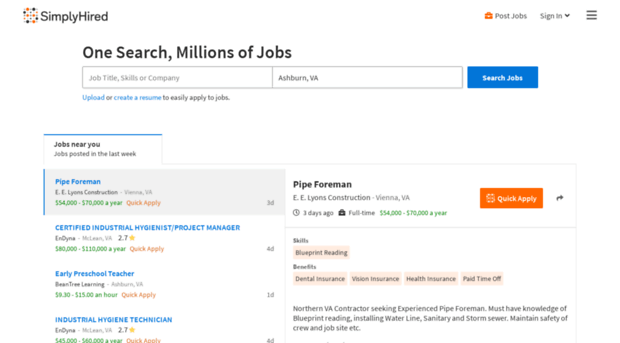This image is a screenshot from the website "Simply Hired." The background of the page is white, giving it a clean and uncluttered look. In the top-left corner, there is a distinctive logo consisting of a square formed by various dots or circles, some of which are black and some are orange. To the right of the logo, the site's name "Simply Hired" is prominently displayed in a straightforward font.

On the far right side of the page, there are two buttons: one for posting jobs and another for signing in to the site. Centered below the header is a bold statement that reads, "One search, millions of jobs," indicating the main utility of the website.

Below this tagline are two input boxes. The first box is intended for the user to input a job title, skills, or company name. To the right of this, a second box allows the user to input a desired location for the job search. Adjacent to these boxes is a blue button labeled "Search Jobs."

Further down, there's a section titled "Jobs Near You," where specific job listings are displayed. Among these listings is a job for a Pipe Foreman, which includes a quick apply button to the right. Beneath the job title, there are key details such as required skills, benefits, pay rate, and the notation that it is a full-time position. Additional job listings are organized below this one, aligned on the left side of the page.